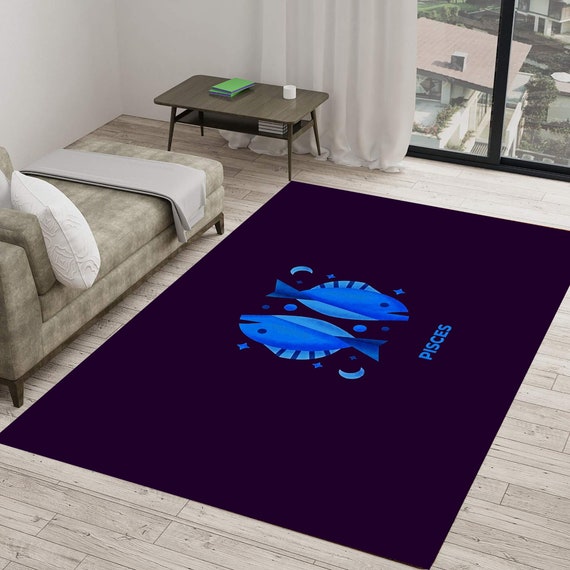The photograph captures a minimalist, modern apartment bathed in natural light from a floor-to-ceiling window with a black frame, partially covered by sheer white full-length curtains. The main focal point is a large, dark blue rug that dominates the center of the room, adorned with an artistic depiction of the Pisces zodiac sign, featuring two light blue fish facing opposite directions amidst two half moons and four stars. To the left, a tan chaise lounge with white pillows and a neatly folded gray blanket rests invitingly, complemented by a mid-century 1960s-style table at its base. The table boasts a glossy brown wood finish and holds a few green and white items, possibly notepads or coasters. The light-colored wood floors and the white walls enhance the room's airy, uncluttered aesthetic, reminiscent of Japanese design. Outside the window, the rooftops of neighboring buildings hint at the apartment's elevated position, adding a casual urban charm to the serene interior.